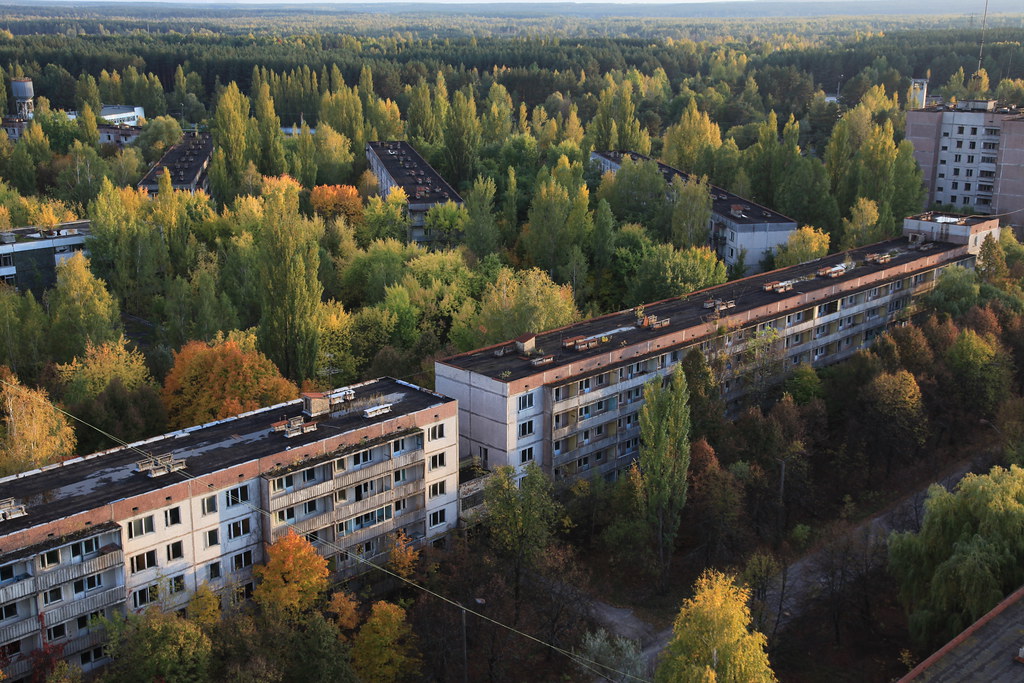The image presents an overhead view of a town or city dominated by an expansive, verdant landscape of mostly green trees extending into the distance, dotted with patches of orange and yellow foliage indicating the onset of fall. Two prominent, long rectangular apartment buildings, aligned diagonally from the bottom left to the top right corner, stand out amidst this sea of greenery. These buildings, characterized by their white brick facades and black roofs with numerous balconies, appear neglected, with dirt-covered and deteriorating features. Several other similar structures are scattered throughout the scene, surrounded by dense clusters of trees, particularly thick at the image's top and bottom. Among the trees and buildings, various roads and driveways are visible, weaving through the landscape.